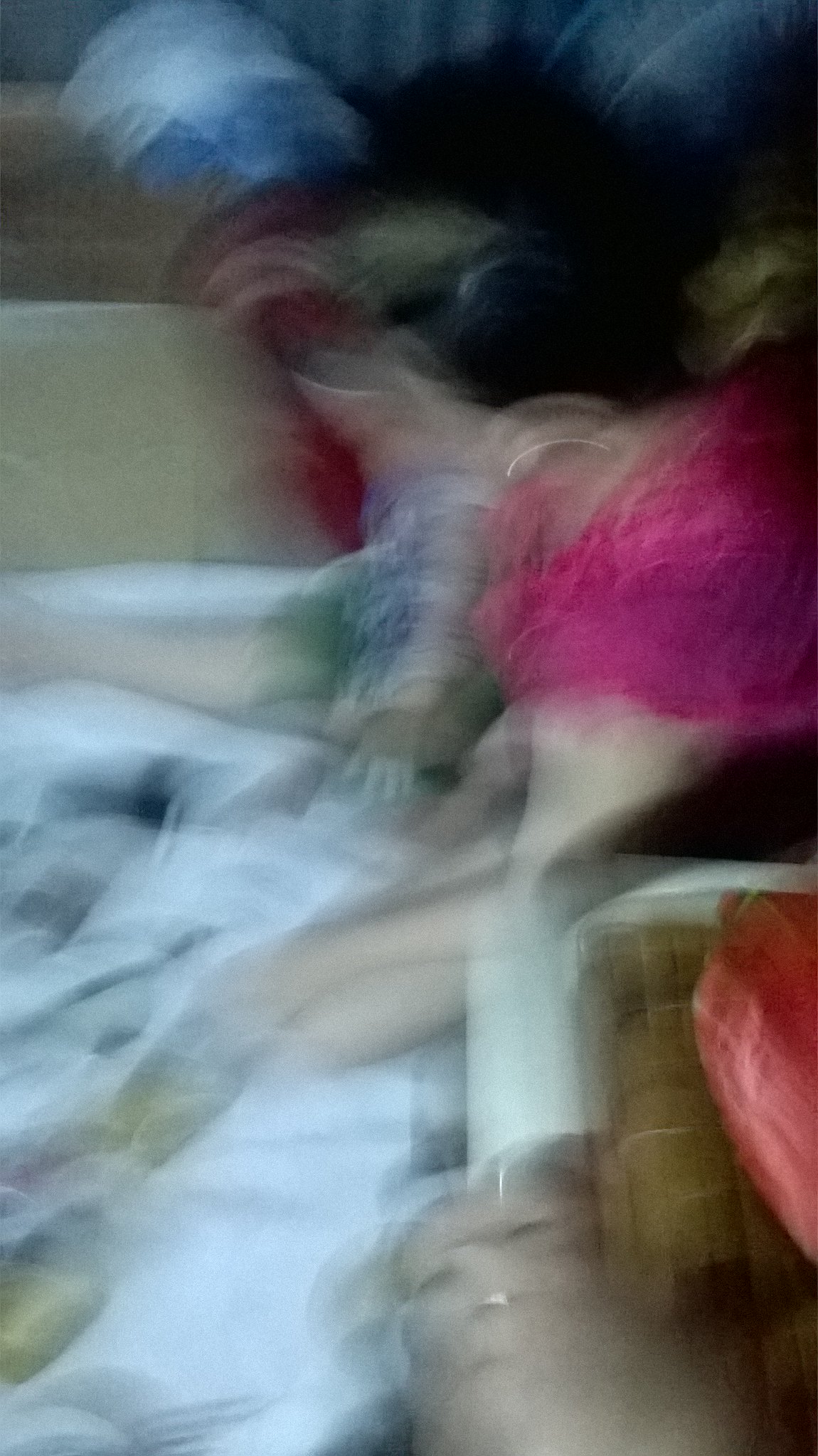The image is highly blurry and distorted, making it challenging to decipher specific details. At the top, there are faint outlines of two individuals seated side by side. One appears to be a woman wearing a pink top, with legs extending towards the left. Next to her, there might be another woman with red hair, although this is difficult to confirm due to the poor quality of the image. The background behind them features a greyish surface with hints of blue at the top.

In the bottom section of the image, there is a fragmented and distorted face of a woman with light-colored hair. Her facial features, including the eyes and nose, are somewhat visible, but the right side of her mouth is heavily blurred. This distorted face appears beneath a chaotic overlay of objects, including what seems to be a brown box and a pink box on the right side. To the left, there is a large item that resembles either a menu or a piece of paper with designs on it, with white elements superimposed over the entire scene.